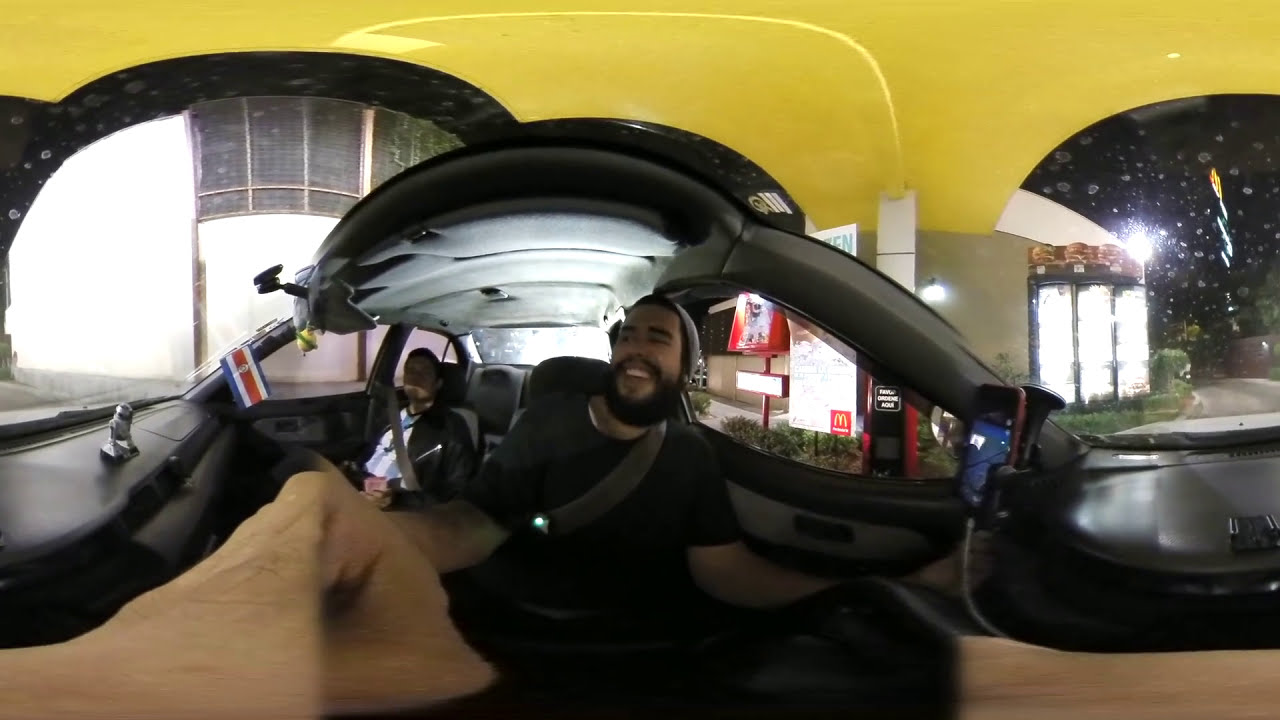The image displays a night-time scene inside a yellow sports car navigating through a McDonald's drive-thru. The photograph appears distorted, resembling a 360-degree video unfurled, causing the subjects and objects to appear elongated and warped. The driver, a dark-complected man with a thick black beard and mustache, is wearing a gray beanie and a black t-shirt. His hand, holding the camera, is visibly stretched due to the image distortion. The passenger, harder to see due to his position farther from the camera, is clad in a white shirt with a black leather jacket. Both individuals are wearing seatbelts. The car's interior features a black dashboard and doors with a black top and gray trim on the sides. In the background, McDonald's branding is visible, including a sign with the foreign text "ORDENE AQUI" indicating the drive-thru order point. A flag inside the vehicle displays a blue background with white and red elements. Additional details such as a yellow object hanging from the passenger side mirror can be discerned, contributing to the overall intricacy of the scene.